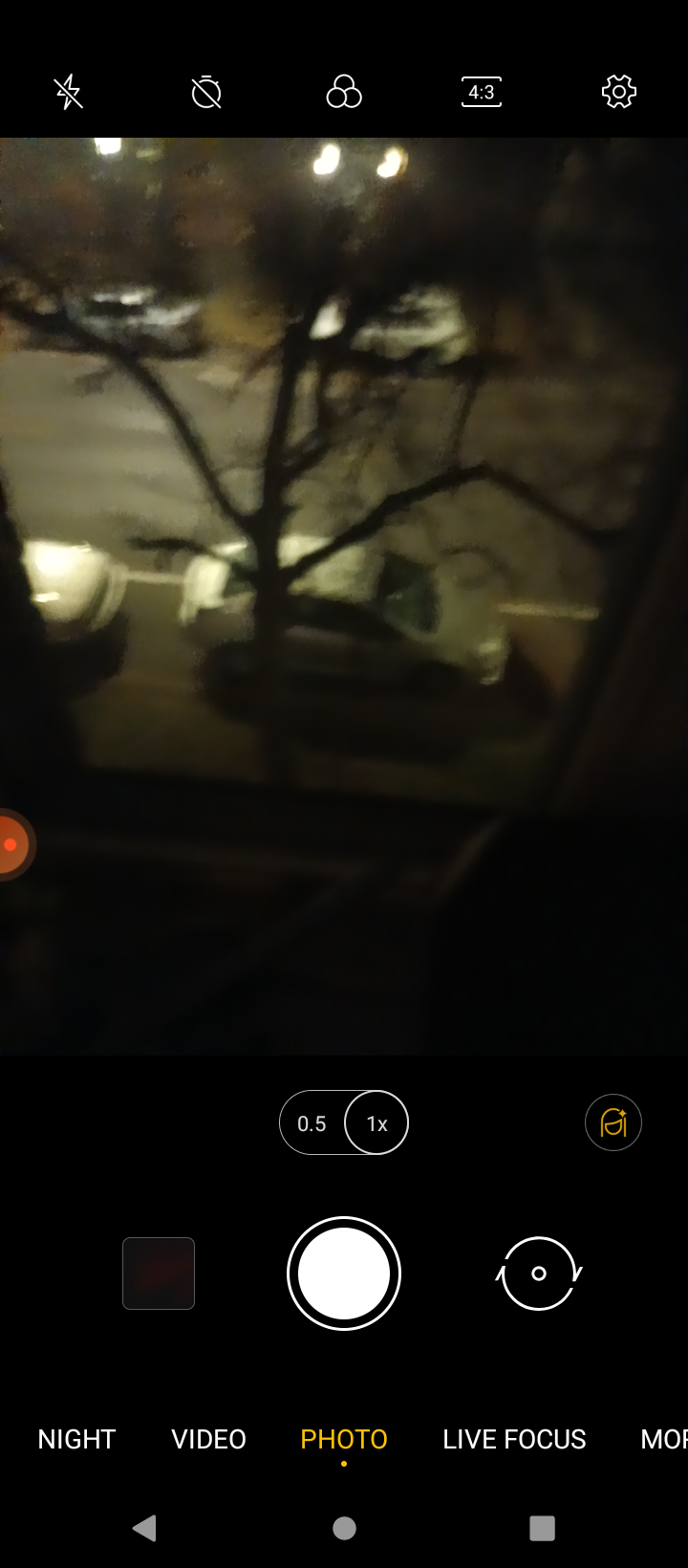This image is a detailed screenshot captured on a phone's camera app. The interface clearly displays the standard camera app features, with black bars at the top and bottom. The top bar includes five icons: a lightning bolt for flash, a circle with a diagonal dash indicating no flash, three concentric circles, “4:3” for aspect ratio, and a gear symbol for settings. The bottom bar shows menu options such as Night, Video, Photo, and Live Focus, with the Photo mode currently active, indicated by yellow-highlighted text. The prominent white button at the bottom is designed for taking pictures, alongside a swirly arrow icon for flipping the camera.

The central part of the screenshot, which takes up about 60% of the frame, displays the camera's view looking down from what appears to be a balcony or an apartment window. The scene captures a street below, where a large tree stands prominently in the center. The tree is surrounded by four vehicles: two are parked close to the viewing point and are silver in color, while the other two vehicles are farther across the street, one white and the other a darker creamy white. The street itself is asphalt black, bordered by a gray sidewalk at the bottom part of the image. The clear distinction between different elements within the camera app interface and the outdoor view makes this a well-detailed and descriptive screenshot.